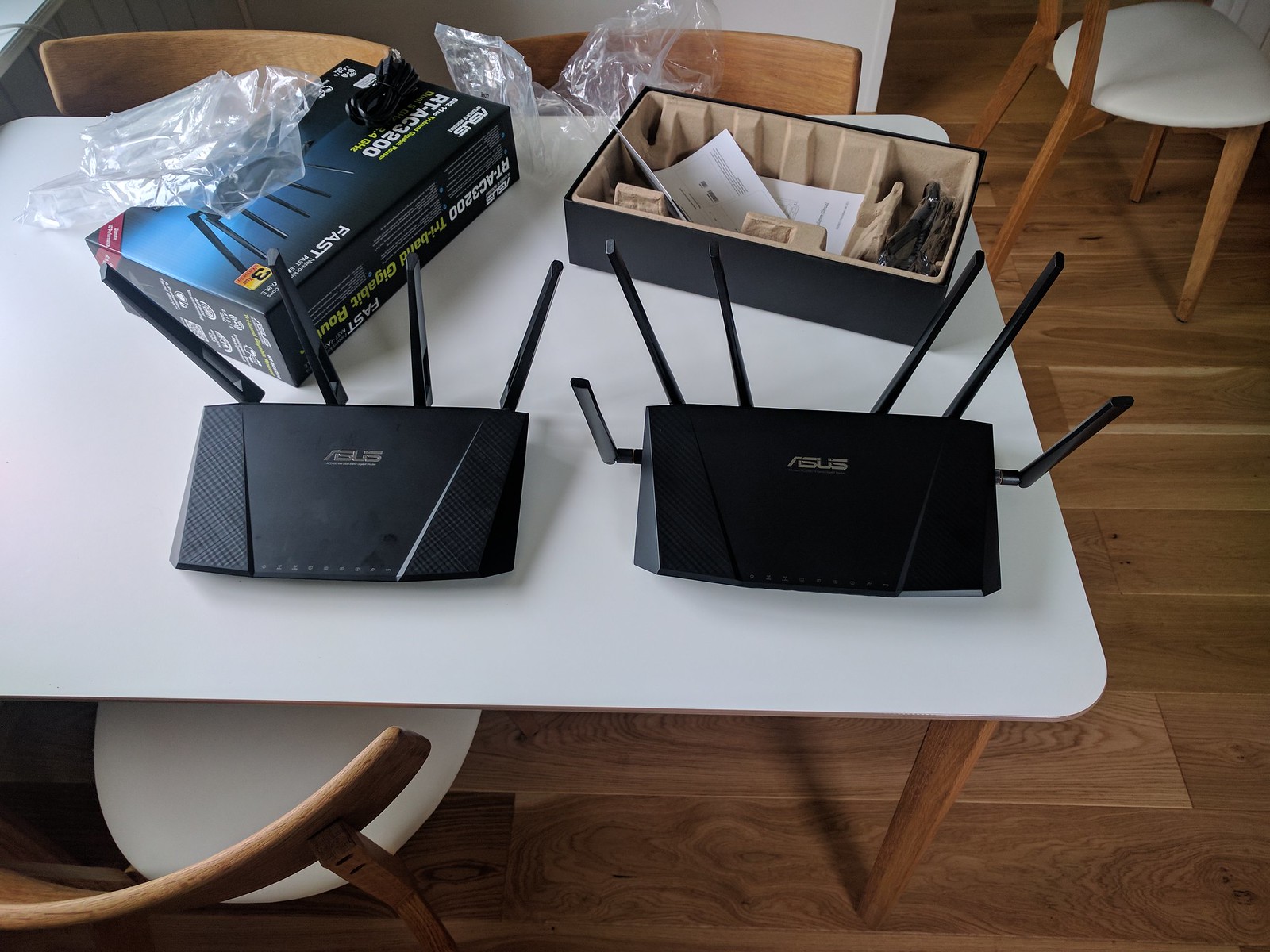The image showcases a setup with two Asus Wi-Fi routers prominently displayed on a simple white table. The table, oriented horizontally in the image, has light brown wooden legs. The surrounding area features light brown paneled wood flooring, contributing to a warm atmosphere. There are multiple chairs depicted: one in the bottom left corner with an off-white cushion and light brown wooden legs, and another on the upper part of the table showing its curved brown back. Additionally, there is a chair in the top right corner, facing towards the right, with similar wooden legs and a white cushion.

On the table, two Asus routers stand out. The router on the right has six tall antennas—four at the back, one on the right, and one on the left. The router on the left has four antennas positioned at the back. Behind the routers, a black packaging box with white text reads "FAST" and "ASUS" on the left. The box, partially open, reveals a brown interior and a white manual paper. To the left of these items, there is another packaging box labeled "RTAC3200" in white text along with "Tri-Band Gigabit Router" in green. This box is similarly marked with "FAST" at the top. Clear plastic and a black cord are also visible on the white table surface. The scene is framed against a plain white wall, emphasizing the clean and organized display of the computer equipment.